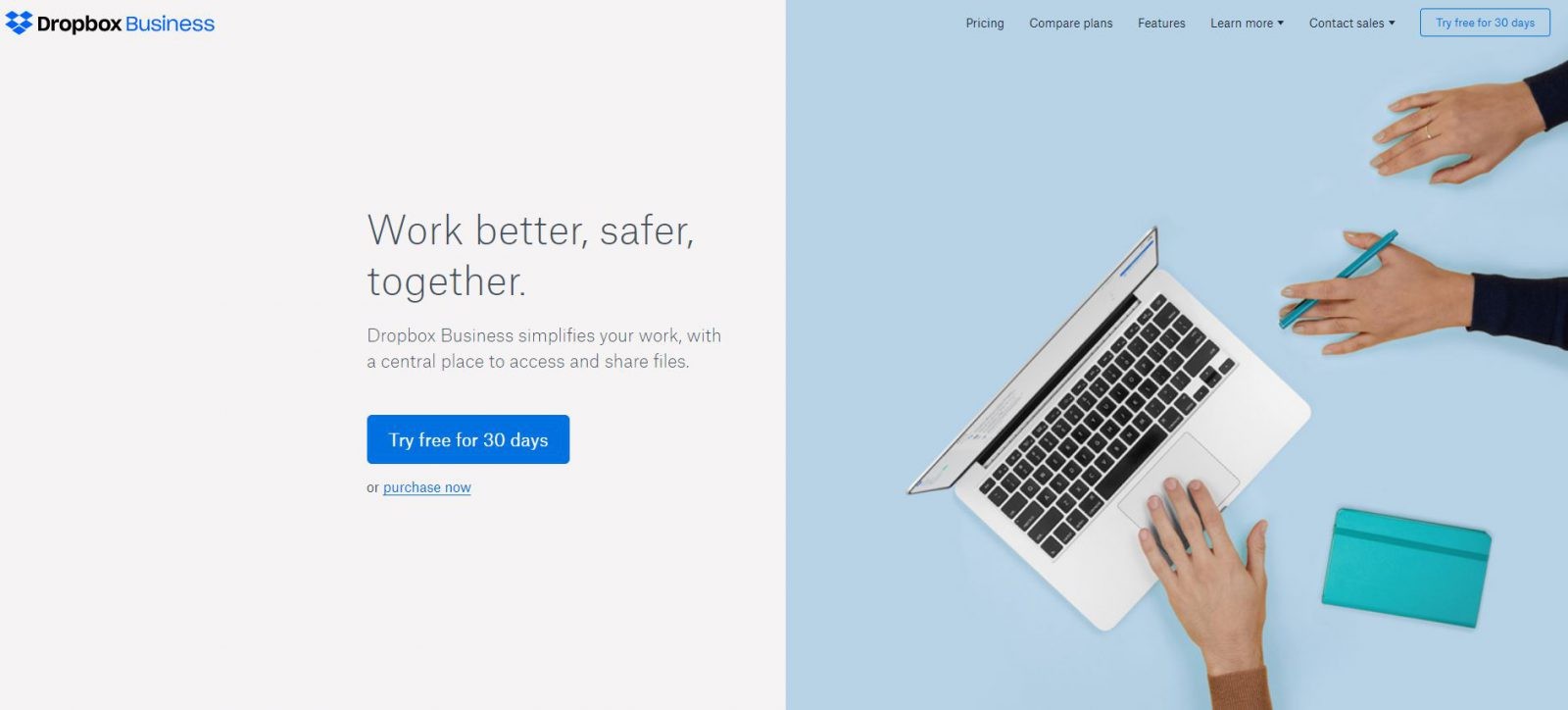The image showcases a professional website interface for Dropbox Business, emphasizing its features designed to streamline work by offering straightforward access and sharing of files. Central to the image is a prominent blue rectangle with the text "Try Free for 30 Days or Purchase Now." The top right corner displays navigation options including "Pricing," "Compare Plans," "Features," "Learn More," "Contact Sales," and "Try Free for 30 Days."

In the background, the setup includes a blue table and a light blue mat. On the right side of the image, a person dressed in a black sweater is visible, with their right hand's middle finger adorned with a ring. They are holding a pen in their left hand, and a hint of a brown sweater is visible at the bottom portion. To the immediate right at the bottom, there is a light blue journal and a strap, adjacent to a silver MacBook laptop with a thin screen, black hinge, and black keys. Overall, the imagery captures a clean, professional environment highlighting the user-friendly interface and cohesive design of the Dropbox Business website.